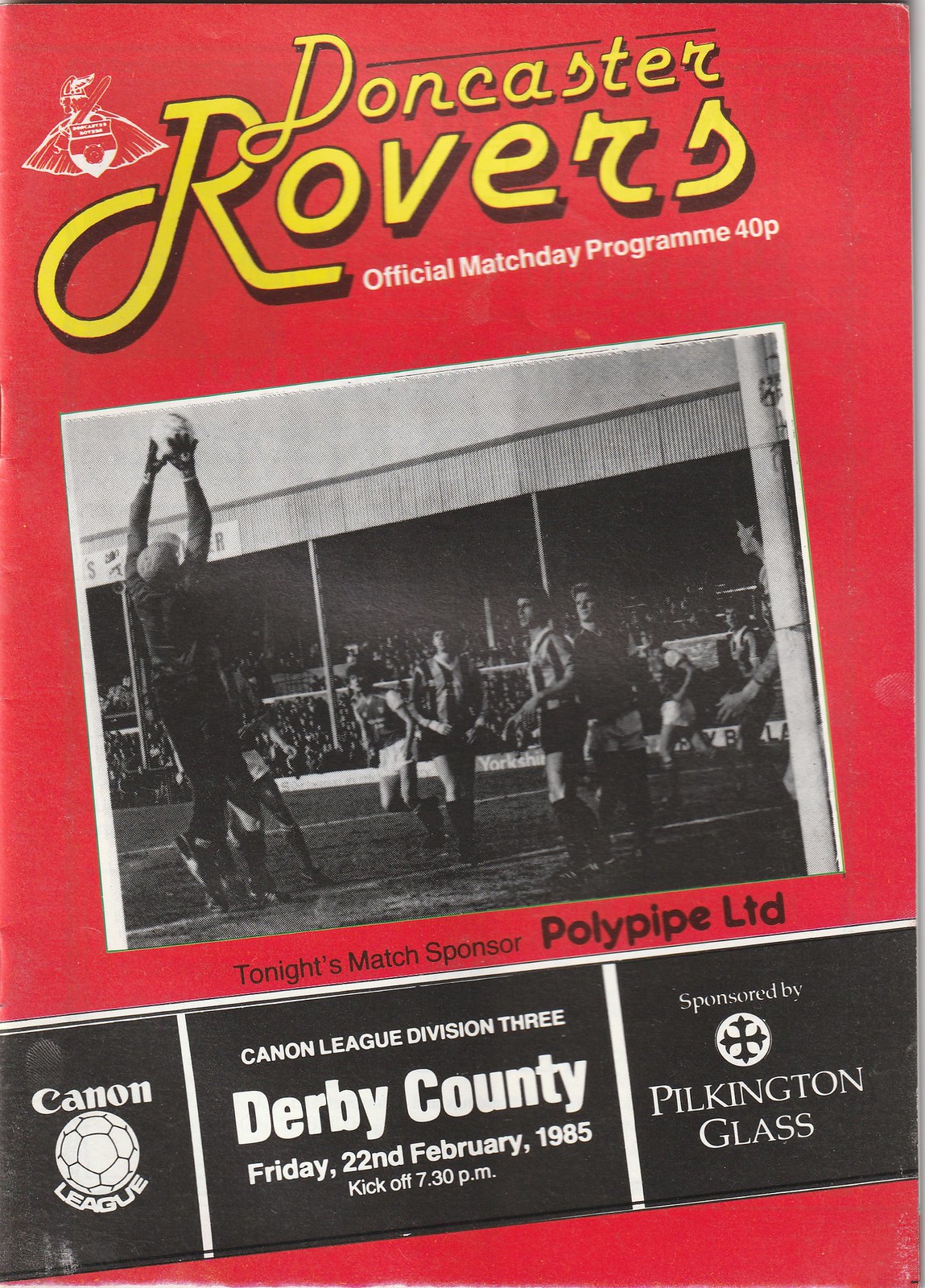This is the cover of an official soccer match program for Doncaster Rovers. The background is entirely red, and at the top, in a disjointed, retro-style yellow script, it reads “Doncaster Rovers.” Below this, in smaller white text, it says “Official Match Day Program 40P,” slanted diagonally upward from left to right. A black and white photo beneath the text features a dramatic moment from a game showing a goalie jumping with both hands outstretched to block a soccer ball, with a backdrop of a crowded stadium. Under the photo, "Tonight's Match Sponsor Polypipe Limited" is printed in bold black lettering. At the bottom of the cover, a black bar outlined in white is divided into three sections. The left section displays the Canon League logo with a white soccer ball. The middle section reads "Canon League Division III" at the top, followed by "Derby County" in large text, and "Friday, 22nd February 1985, Kickoff 7.30 p.m." in smaller white text. The right section contains a smaller logo of Pilkington Glass, consisting of a circle with a double cross in the center, and the text "Sponsored by Pilkington Glass."